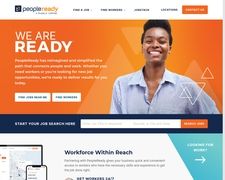This screenshot captures an advertisement on the People Ready website. Prominent at the top left corner is the website's logo. The focal point is a large, vibrant banner in the center, predominantly showcasing the slogan "We Are Ready" boldly positioned on the left side. The right side of the banner features a young Black man, likely in his early 20s or younger. He is smiling warmly and dressed in a blue button-down shirt. The ad features a dynamic color palette, incorporating gradients of light, medium, and dark orange, contrasted with light blue and some areas of white.

Directly beneath this main advertisement banner is a navy blue section that includes a search bar for user interaction. Below this, there is additional text stating "Workforce Within Reach," emphasizing People Ready's mission. At the very top of the screenshot, there are two small buttons, though their specific functions are not discernible. This detailed depiction highlights the use of color and layout employed by People Ready to convey their branding and message effectively.